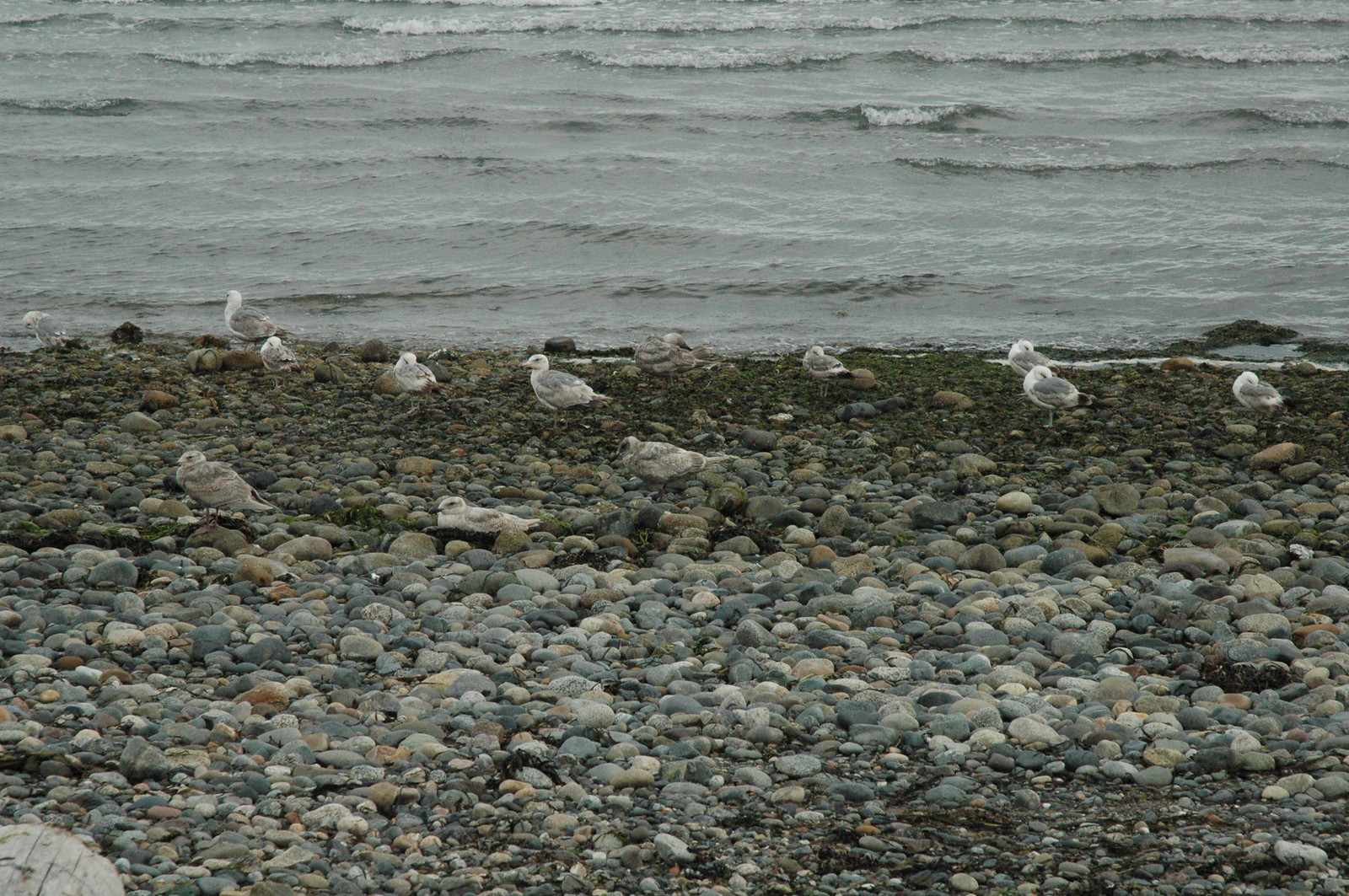This photograph captures a wide, rocky beach with no sand, just an array of rocks varying from gravel to fist-sized stones. Scattered along the shore, closer to the water, are at least thirteen seabirds, likely terns, with varying amounts of gray and white in their plumage. The majority have gray wings and white necks and heads, though a few are almost entirely gray, and some display more white in the neck. Many of the birds appear to be resting, with their heads tucked into their feathers. The background features a body of water with small waves approaching the shore, and hints of greenery, possibly moss, line the water's edge. Additionally, parts of a log can be seen in the lower right and left corners of the image.